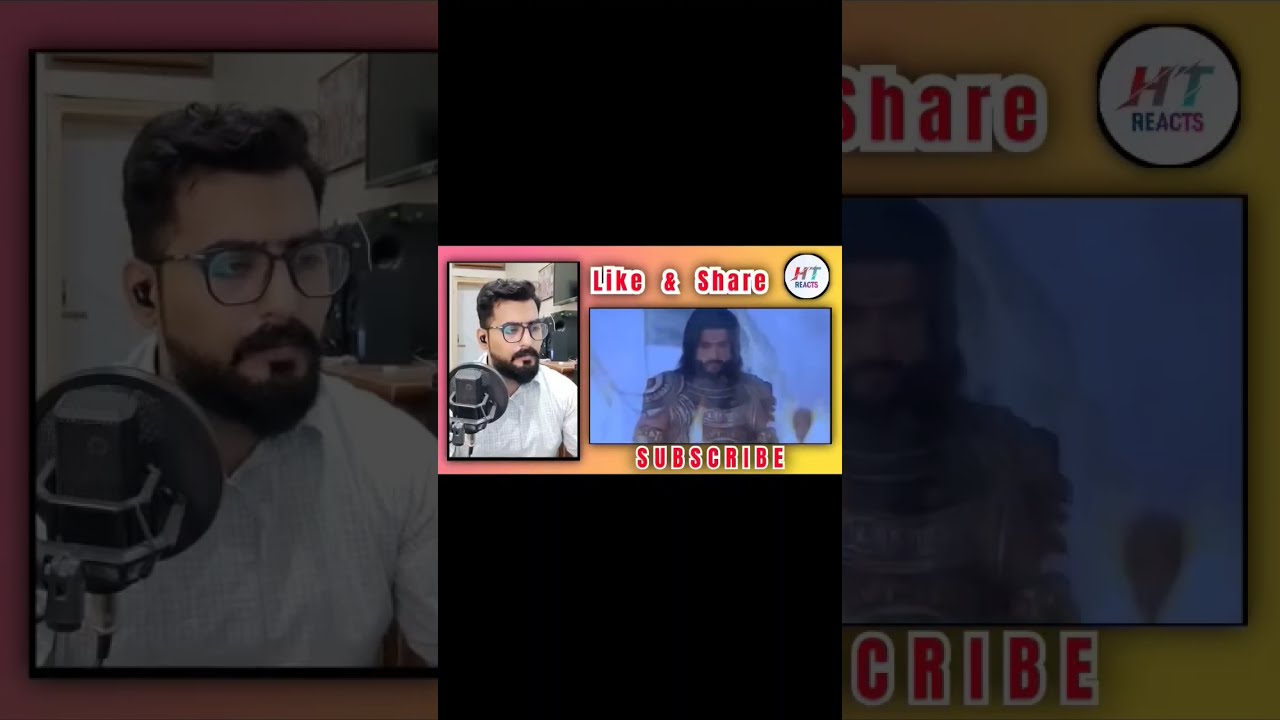The image is a small, inset color photo set against a larger, darkened background. It depicts two video screenshots side by side, resembling a YouTube video or podcast. On the left is a man in a recording studio, wearing a white shirt and black eyeglasses, with a dark beard and hair. He is speaking into a round microphone. To the right is an interviewee or performer with long dark hair, a beard and mustache, dressed in a jacket with a possible design, standing in front of a blue background that includes white curtains. The text overlaid on the inset includes "Like and Share" at the top in a red and white font, and "Subscribe" at the bottom in the same style. In the top right corner, a circular logo reads "HT Reacts," with "HT" in multicolored italic font and "Reacts" in black type. The image captures a freeze-frame of an engaging broadcast session.